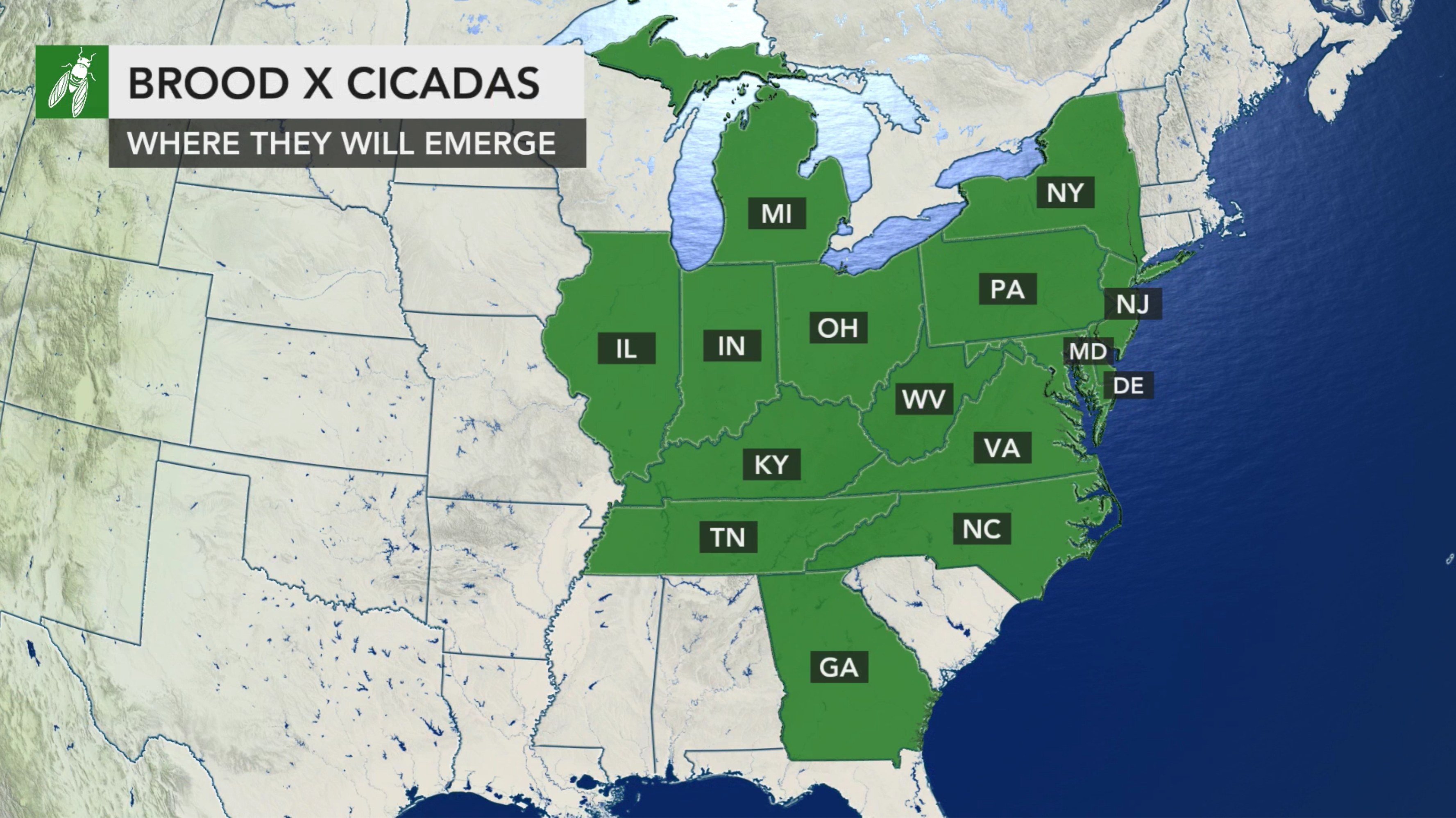This detailed illustration showcases a map of the United States, focusing on the eastern and midwestern regions, with several states highlighted in green. The highlighted states – Georgia, Tennessee, North Carolina, Kentucky, Virginia, West Virginia, Ohio, Indiana, Illinois, Michigan, Pennsylvania, New York, New Jersey, Maryland, and Delaware – are marked to indicate the emergence of Brood X cicadas. These states are contiguous to each other and have their initials displayed in white ticks over black squares. A legend located at the top left of the map indicates that green denotes the areas where the cicadas will emerge, accompanied by a small green cicada icon. While the rest of the map remains a tan or whitish color, the Great Lakes are vividly colored blue, enhancing the visual distinction between affected and unaffected areas.